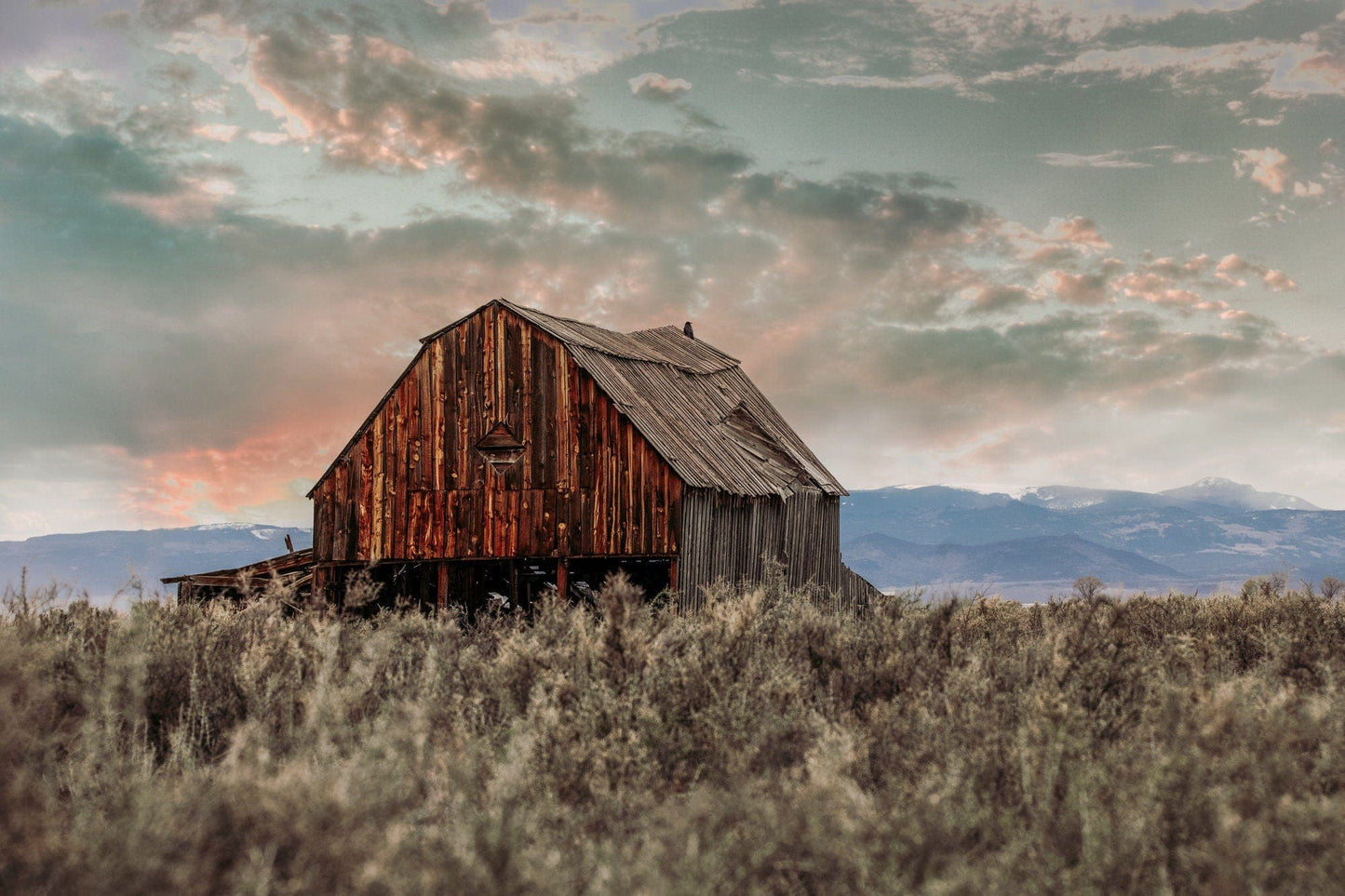In this outdoor photograph, the lower portion features a field of high, dry grass interspersed with small plants, displaying various shades of grey and white, suggesting a muted, almost monochromatic palette. Centrally positioned in this field, there's an old wooden structure that seems to be a house or possibly a barn. The building is brown with a patched, triangular wooden roof, appearing aged and weathered with parts of it a greyish color. Behind this wooden house, a distant mountain range extends across the middle of the image. The mountains are tinged with blue hues, indicating their distance. Above, the sky is filled with dramatic clouds in shades of dark grey, red, and white, creating a striking contrast against the rest of the scene. The overall lighting suggests a dusky or early evening setting, enhancing the image's atmospheric quality. No people, words, or numbers are present, allowing the natural and architectural elements to stand out clearly.